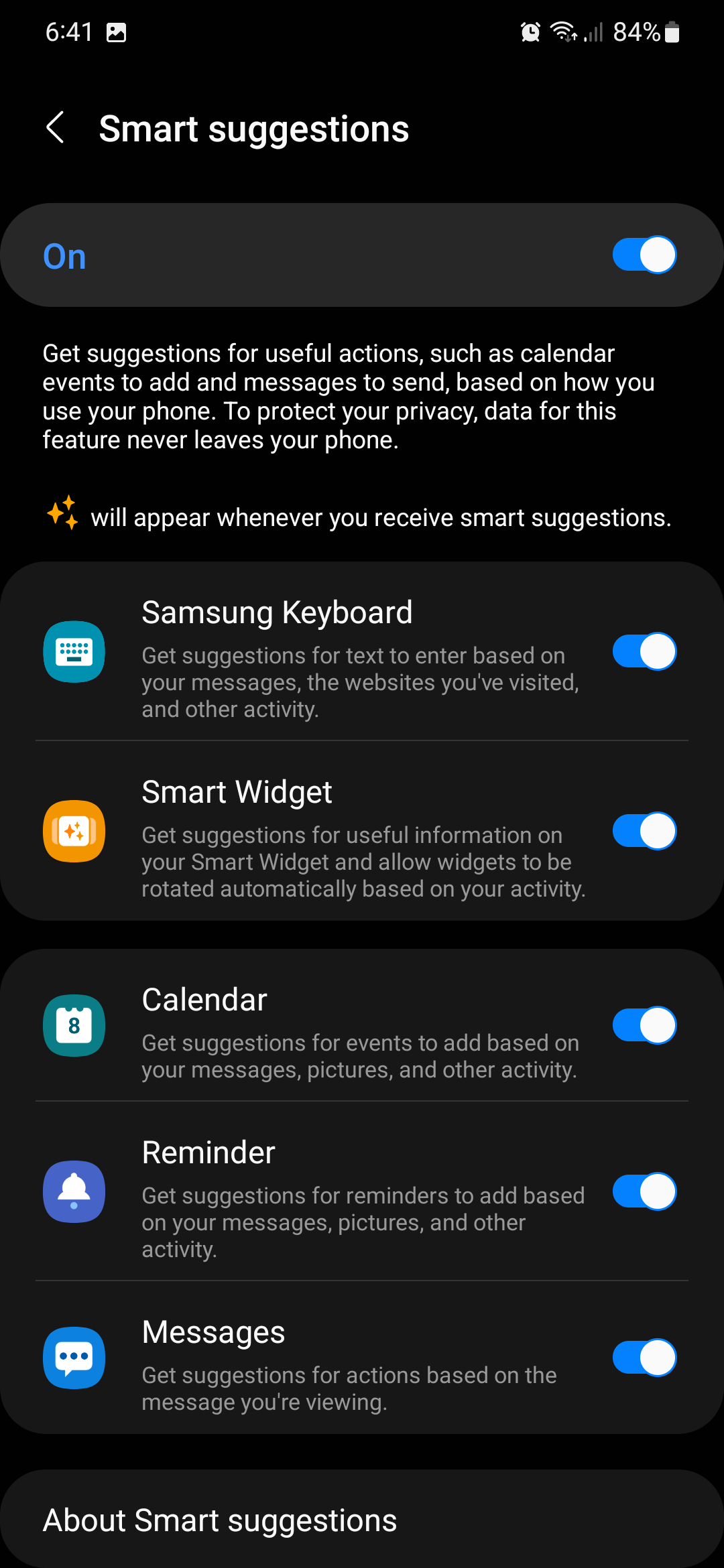In this detailed screenshot of an Android device, several elements and settings are prominently featured. The screenshot highlights the "Smart Suggestions" functionality, which provides useful action suggestions such as adding calendar events and sending messages based on phone usage. This feature emphasizes user privacy, with data processing staying entirely on the device.

The image shows "Smart Suggestions" in various states: Samsung Keyboard is activated, Smart Widgets are on, and Calendar, Reminder, and Messages functionalities are also turned on. 

In the upper left corner of the screenshot, the device time is displayed as 6:41. Additionally, a gallery icon is visible. The status bar includes several icons, indicating that an alarm is active, Wi-Fi is connected, there is a good signal strength, and the battery is at a specific percentage level.